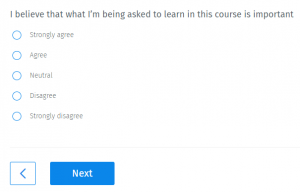This image displays a survey question interface on a white background. At the top, in gray text, it asks, "I believe that what I'm being asked to learn in this course is important." Below the question, there are five outlined blue circles with white interiors arranged vertically. Each circle corresponds to an answer choice, which are listed to the right in gray text. The options, from top to bottom, are: "Strongly Agree," "Agree," "Neutral," "Disagree," and "Strongly Disagree." These circles resemble selection options you might find on a standardized test form, where participants are meant to select one. At the bottom of the image, there is a navigation bar. On the left, there is a white box with a back arrow, allowing users to return to the previous question. To its right, there is a blue rectangular box labeled "Next," which users can click to proceed to the next question. The overall layout is clean and straightforward, with the background remaining completely white.